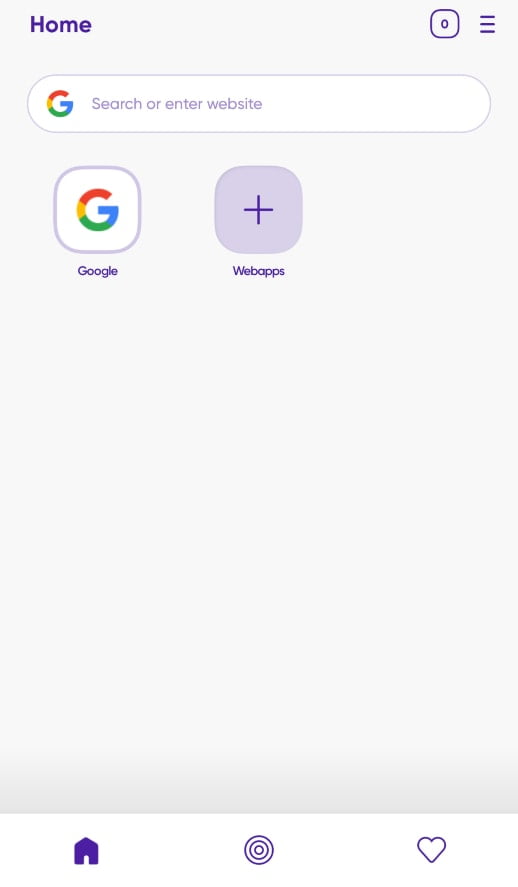This image appears to be a screenshot or mock-up of a mobile interface, predominantly themed in shades of purple and lavender. At the top left corner, there is a purple button labeled "Home." Adjacent to it, on the far right, is a square with rounded corners, outlined in purple, containing the digit '0'. To its immediate right is a purple hamburger menu icon.

Below this, a rectangular area with a lavender outline designated for a Google search is visible, containing the prompt "search or enter website" in lavender text. Directly beneath this search bar, there are two icons: the first is the familiar Google icon featuring the multicolored "G" logo, framed within a square tile with large rounded corners. The second icon, to its right, mirrors the tile shape but is solid lavender with a purple plus sign in the center. Below this icon, the label "web apps" is displayed.

The background of the interface is plain white, with no wallpaper or additional visuals. There is a subtle drop shadow effect at the bottom, suggesting a gradient screen that is otherwise blank. At the very bottom of the screen, there are three navigation options. The first is a solid house icon with an outlined door and pitched roof, representing "Home." The second is a target comprising three concentric circles. The third is an outline of a heart. All these navigation icons are rendered in purple.